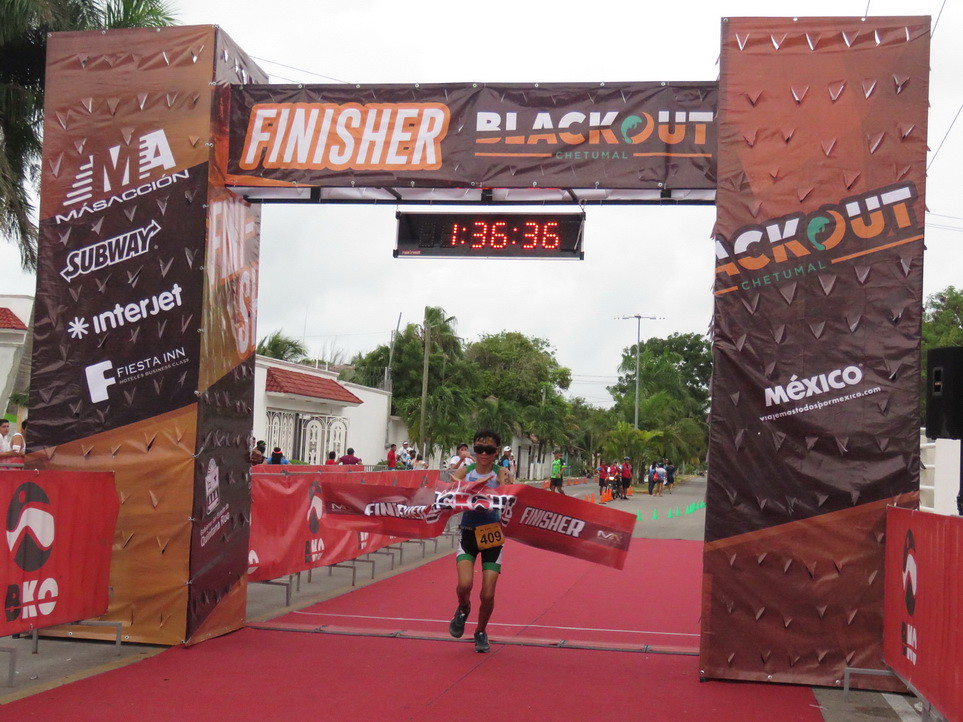The image captures the triumphant moment of a runner crossing the finish line of an outdoor marathon. Dominating the scene is a large, rectangular finish line structure, supported by two tall pillars adorned with various company logos, including Subway, Interjet, and Fiesta Inn. The pillars and a crossbar above the finish line are multi-shaded brown and feature the words "Finisher Blackout" prominently displayed, with a digital clock beneath reading "1:36:36". The runner is breaking through a thick, red tape that repetitively says "Finisher". Spectators are gathered to the left, witnessing the victory, and green cones line the asphalt in the background. The setting is completed by distant trees, power lines overhead, and a red carpet at the finish line, under a pale white sky.